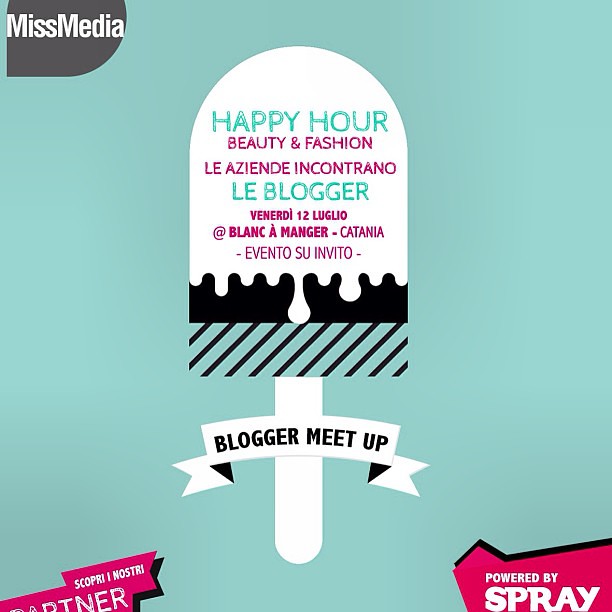This square event advertisement features a background in a light seafoam green hue. In the top left corner, there's a gray circle with a pointed edge that reads "Miss Media" in white font. Central to the image is an illustration that could be interpreted as a popsicle or a microphone shaped like a popsicle; it is primarily white with a black gradient at the bottom and black stripes. Across its stick is a ribbon that reads "Blogger Meetup" in white text. The body of the illustration bears green and red text reading "Happy Hour," "Beauty and Fashion," and additional Italian text detailing the event: "Le aziende incontrano le blogger venerdì 12 luglio at Blanc All Manager Catania. Evento su invito." In the bottom right corner, a bright pink geometric shape with a black shadow above it features the white text "Powered by Spray." Another bright pink shape with white text peeks from the bottom left corner, though the text here is partially obscured.